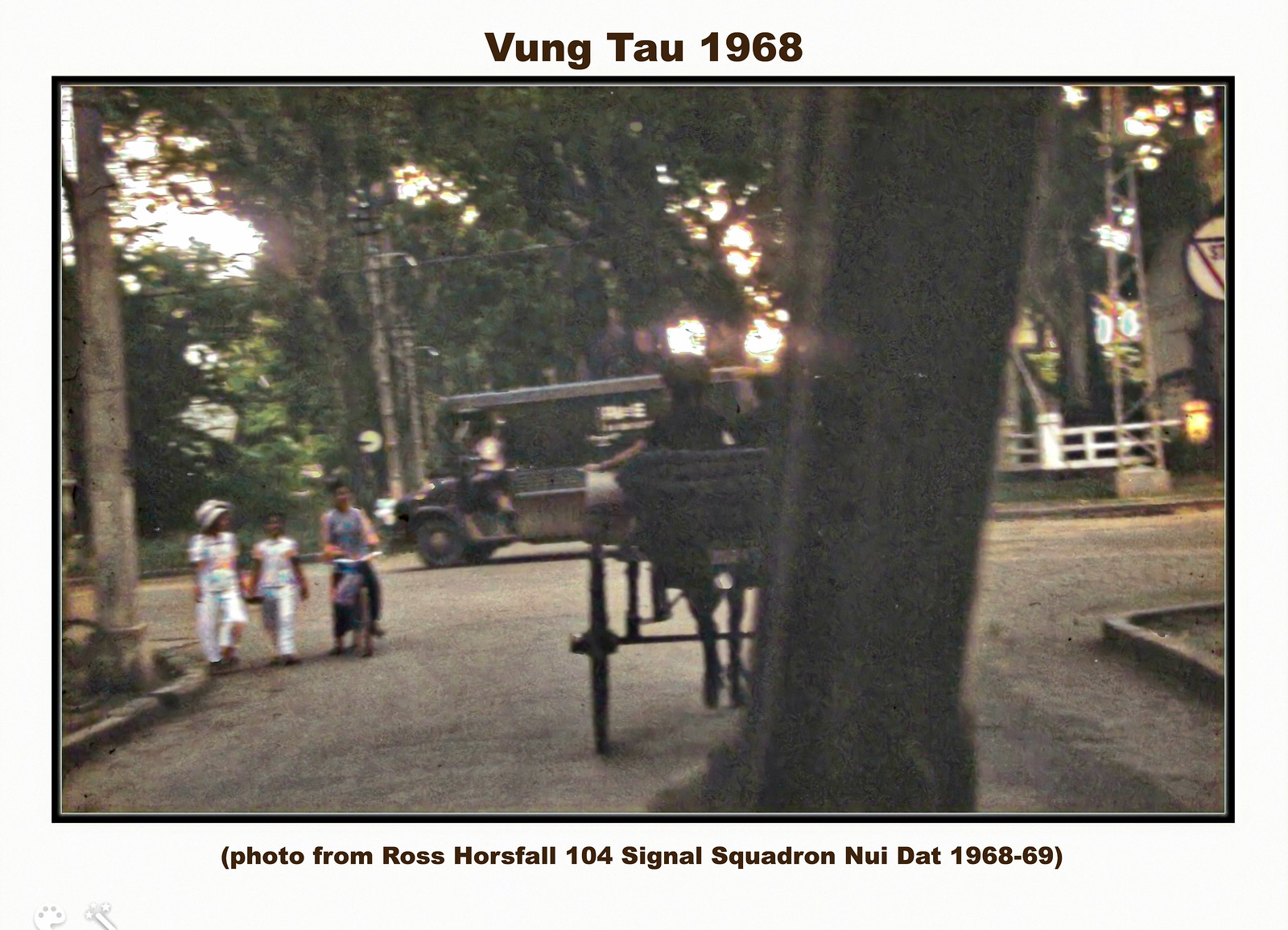The photograph, framed by a white border with a thin black line, has the title "Vung Tau 1968" in bold black letters at the top, and a caption reading "photo from Ross Horsefall, 104 Signal Squadron, Nui Dat 1968-69" in parentheses at the bottom. The image captures a street scene on a dirt road bordered by curbs, possibly taken through the split screen windscreen of a vehicle. At the center of the road, a horse-drawn carriage heads toward the camera, while a panel truck crosses from right to left in front of it. On the left side of the frame, three pedestrians with darker skin tone can be seen: one in a white outfit, another riding a bicycle in a purple outfit, and a third in white. The background reveals a tree-lined scenery and a white fence alongside a gray building, adding depth to this historical snapshot.